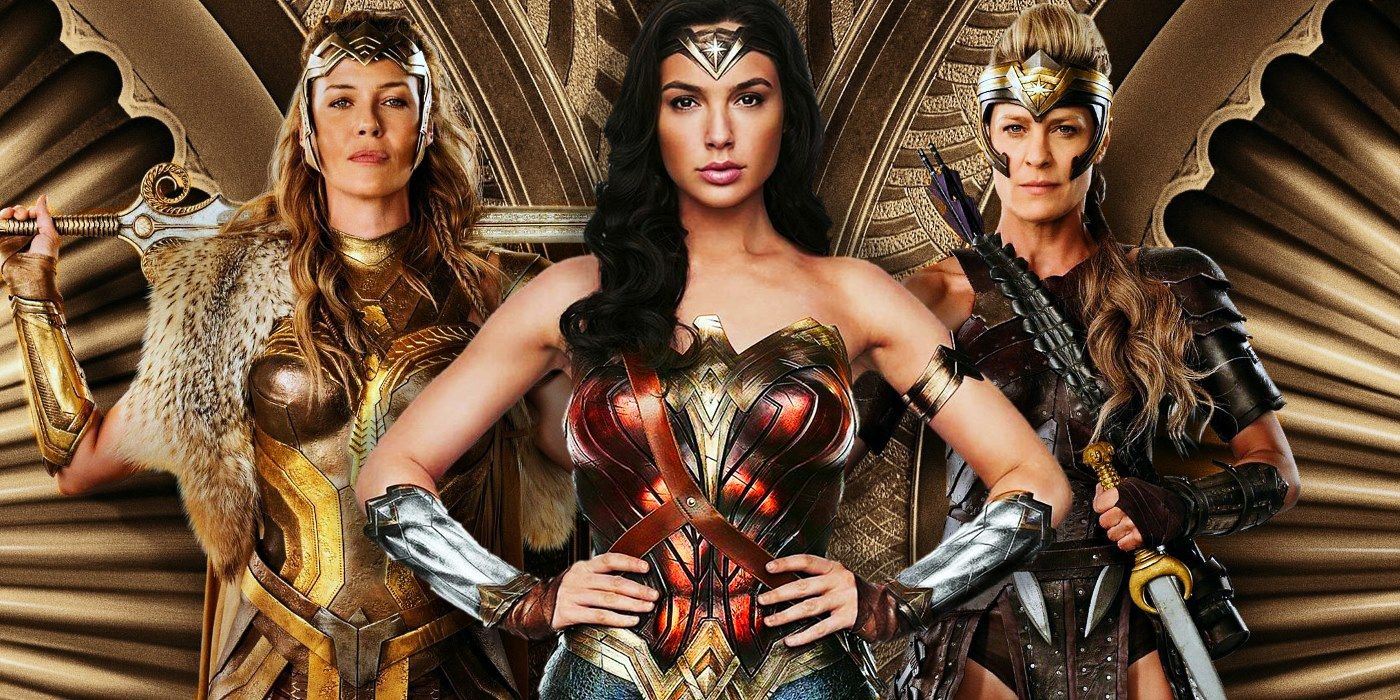In this detailed banner graphic, we see a striking scene featuring three Amazonian warriors from the DC movie franchise, with Wonder Woman positioned prominently at the center. Gal Gadot portrays Wonder Woman, adorned in her iconic red and gold armor, complete with a gold W belt and metal forearm bracers. Her long, wavy black hair frames her determined expression. On either side of her stand two other Amazonian women—one of whom might be Blake Lively—with Robin Wright also identified among them. These two warriors are outfitted in more rugged, brown leather and gold armor, wielding swords and smaller daggers, supplemented by decorative fur elements. The backdrop is a golden, digital landscape with art deco-inspired geometric graphics, enhancing the epic and timeless feel of the image. The trio collectively embodies strength and valor as they pose heroically.